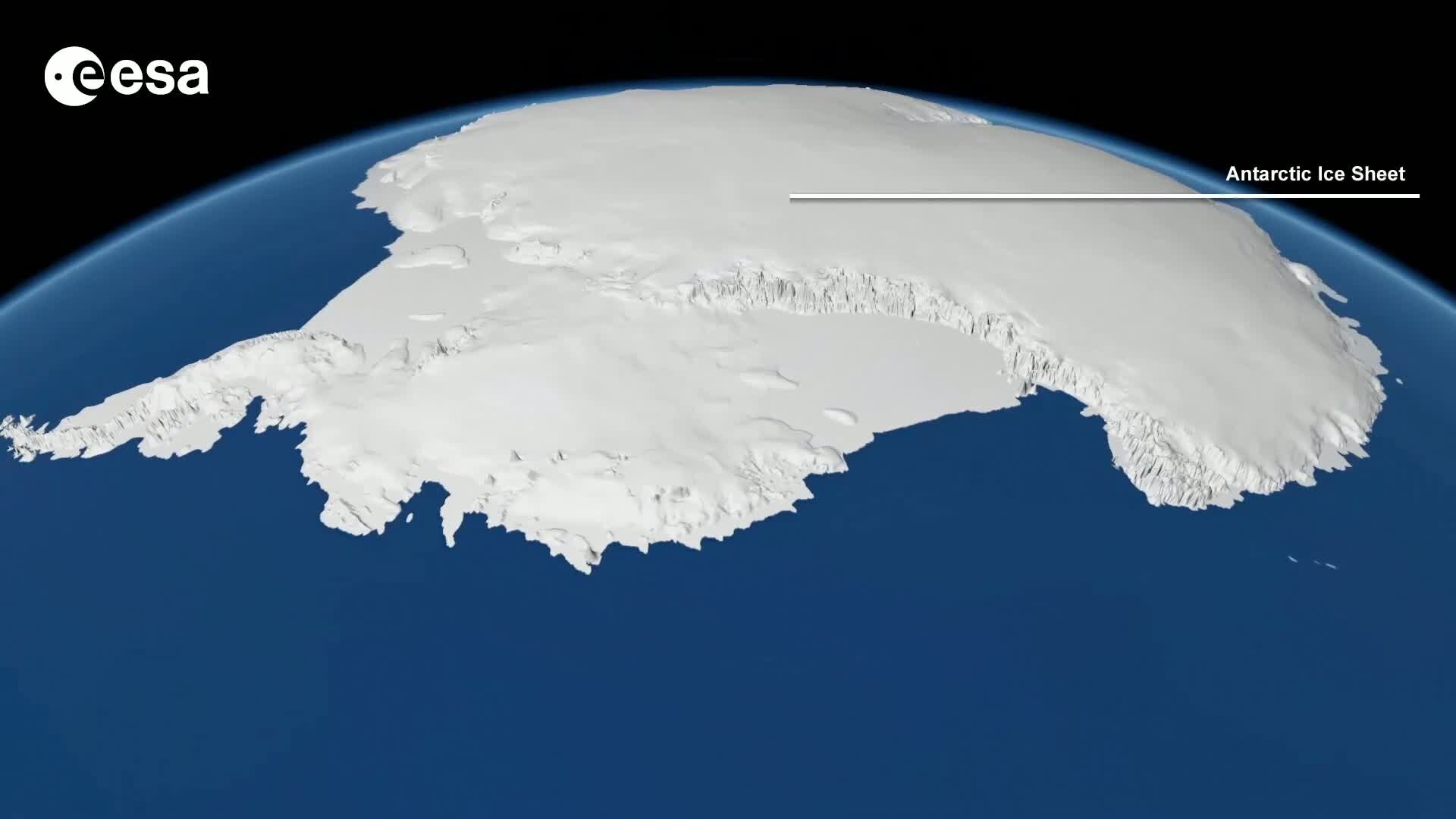The image depicts a digital representation of the Earth, focusing on the Antarctic Ice Sheet. The Earth is colored in a typical blue hue, set against a black background. The upper left corner features the ESA (European Space Agency) logo, with the letter 'E' encircled. The Antarctic Ice Sheet is prominently displayed at the top of the globe, marked by a white, textured expanse that suggests varying thickness, ridges, and hills. A label reading "Antarctic Ice Sheet" points directly to this white region. The ice sheet itself has a distinct, somewhat rounded shape with a tail-like extension on the left, and jagged edges which likely represent the icy boundaries of the glaciers.